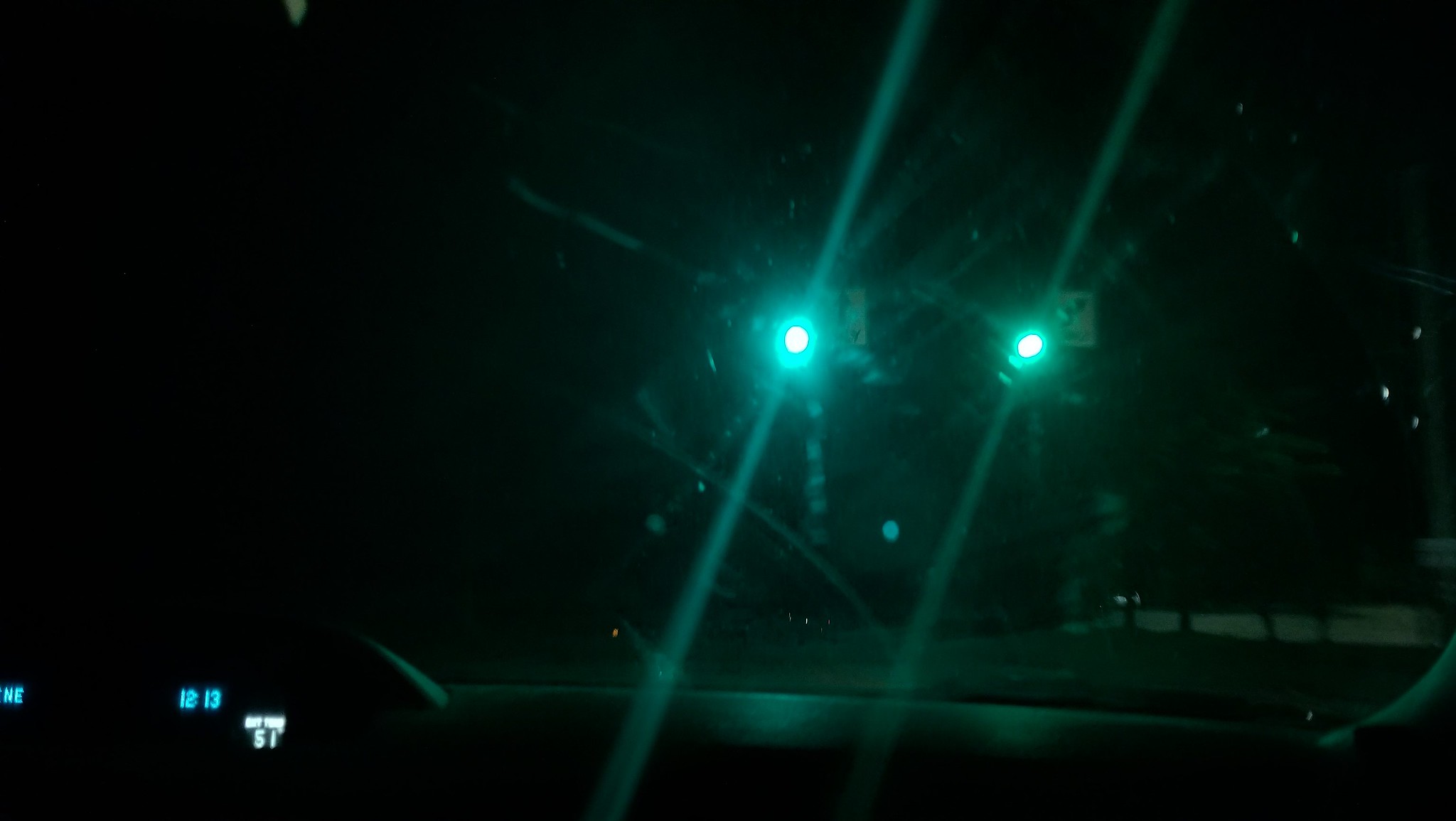A nighttime photograph captures the view from the front seat of a vehicle, looking out through the windshield. At the bottom left of the image, the illuminated green LED on the dashboard reads '12:13,' indicating the time, while the number '51' in white on the right side might suggest the car’s speed. The vehicle's interior, including the dashboard curving downward and extending horizontally, occupies the lower portion of the image. 

Through the windshield, two bright green, almost teal, traffic lights appear heavily overexposed, with diagonal light flares extending from them across the image. These flares create streaks that stretch both upwards and downwards, disappearing out of the frame. Faint outlines of street signs and guardrails can be seen through the lights, with some greenery like grass and hints of trees visible in the dim background. The far right and upper left corners of the image are enveloped in shadow, adding to the nighttime ambiance.